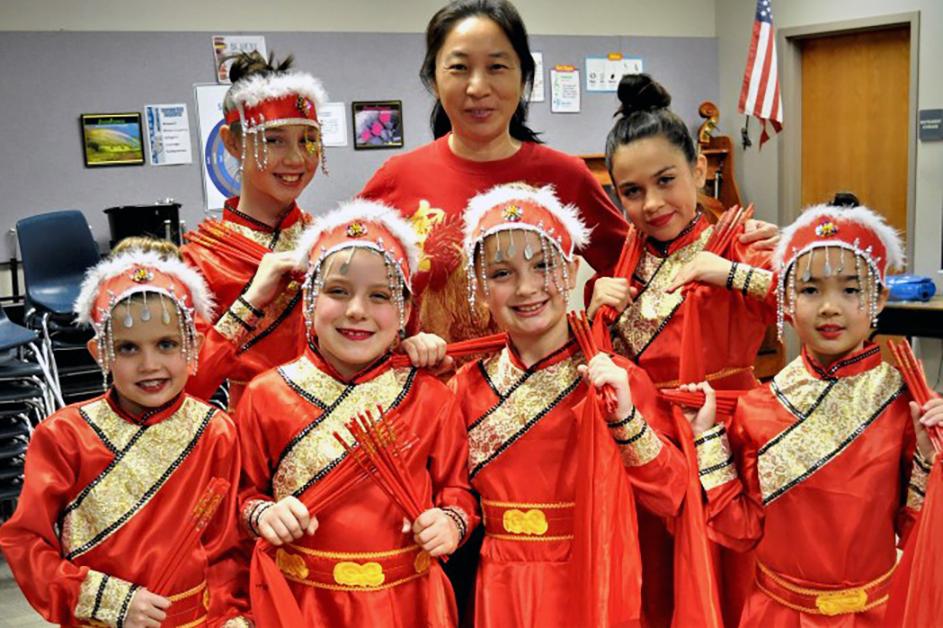In this indoor photograph, a group of six middle-school-aged children is dressed in red costumes that appear to be of Asian design, each adorned with a gold sash featuring intricate gold patterns that might represent dragons or clouds. They hold red sticks or straws with gold writing, further accentuating their traditional look. Each child, except for the girl positioned at the farthest top right, wears a red headband with a white feathery trim, and some also have additional jewelry. Standing at the top center of the group, an older woman with long black hair, dressed in a red T-shirt with a partially visible gold emblem, seems to be their teacher. The setting is a school room, evident from the stacked blue chairs to the left and the American flag to the right, all against a backdrop of plain gray walls.